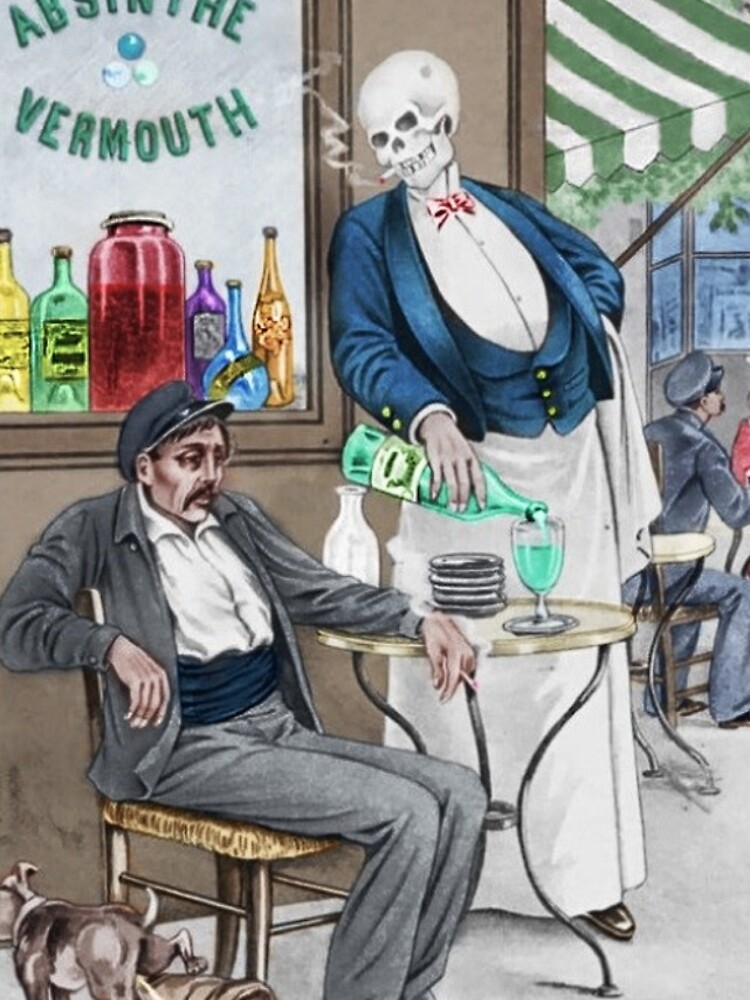The image is a painting or print depicting a striking and surreal scene. A skeleton, identified as a female bartender, is at the center, adorned in a blue jacket, white shirt, red or pink bow tie, and a long white skirt. With a cigarette between its lips, the skeleton is pouring a green liquid, likely absinthe, from a green bottle into a wine glass. The setting appears to be a bar, with a man sitting at a table in a grey suit and hat. The man looks sickly and grey, contrasted starkly by the presence of a small dog at the bottom left of the image. Behind the man, there's a green-and-white striped awning and a window filled with various colorful bottles of liquid, including yellow, green, red, purple, blue, and amber hues. The window bears the partial inscription "ABSINTH E vermouth," hinting at an absinthe establishment. In the background, a police officer is faintly visible, seated and probably keeping a watchful eye on the scene. The painting captures a peculiar and haunting atmosphere, blending elements of fantasy and reality.